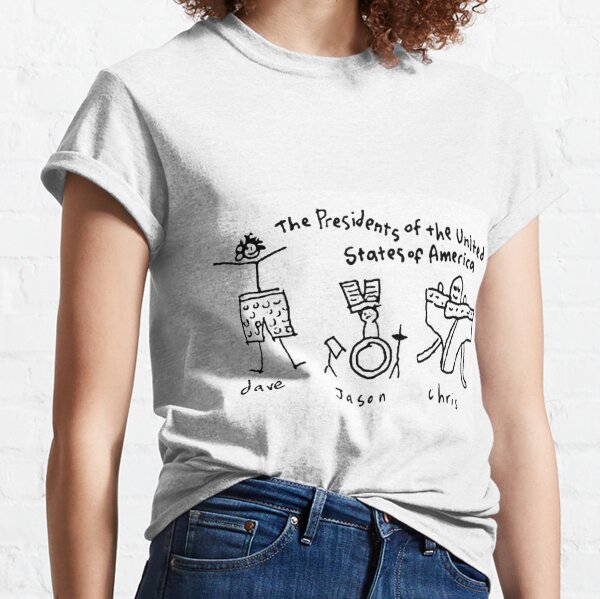The image shows a female with long, curly, reddish hair and fair skin, dressed in a quirky, playful outfit. She is wearing blue jeans, cropped at the waist in the picture, and a white cotton T-shirt with its sleeves rolled up. The shirt is adorned with child-like drawings and handwriting, showcasing three stick figures meant to represent members of the band "Presidents of the United States of America." The text on the shirt reads "The Presidents of the United States of America" and introduces the band members: Dave, depicted wearing only polka dot shorts; Jason, shown behind a drum set with pants on his head; and Chris, covered in briefs, making the figures appear with amusing, whimsical expressions. Her T-shirt is half-tucked into her blue jeans, and her arms are relaxed at her sides.